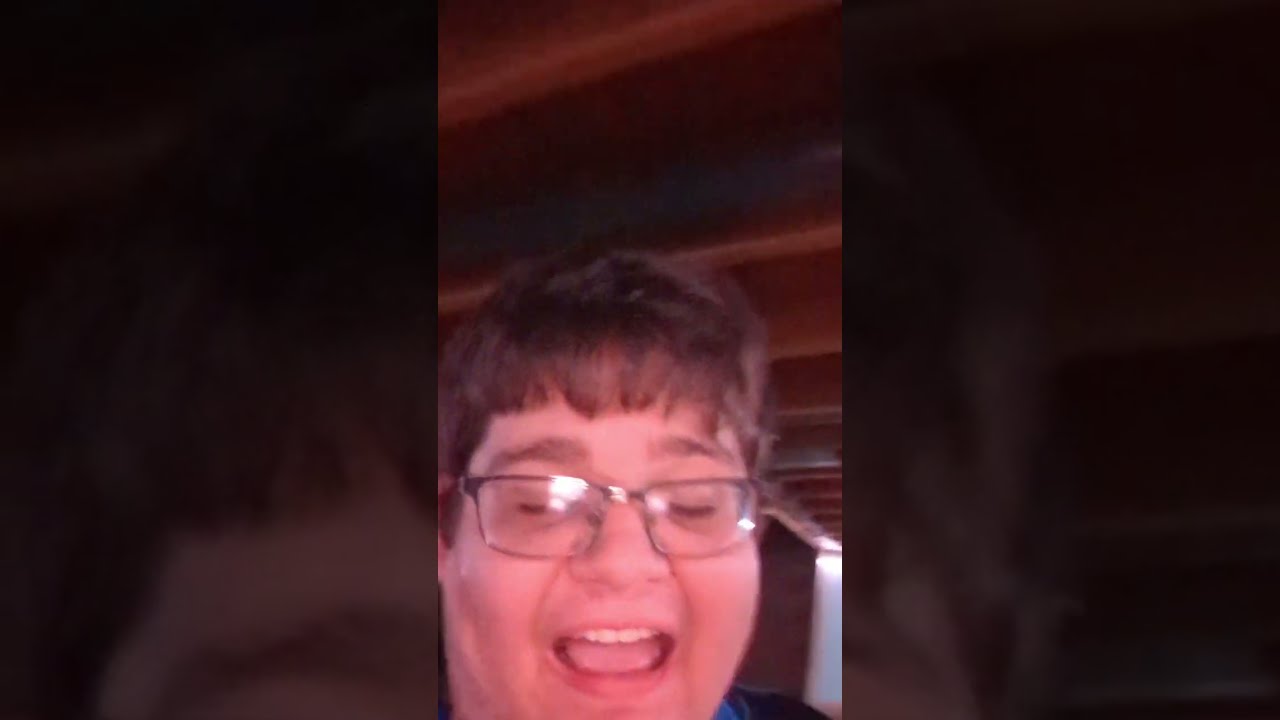The image features a close-up of a Caucasian person with short brown hair and brown eyebrows, set against a dark backdrop divided into three sections. The left and right sections are in shadow, rendering the contents within them indiscernible. In the well-lit central section, the person's face is prominently displayed. They are wearing silver glasses with clear lenses and appear to be in their 40s. Their eyes are closed and they have a broad, joyful smile, with cheeks puffed out, revealing their top teeth and tongue. The photograph captures them from a slightly lower angle, making the wooden rafters of the ceiling visible above their head. There is also a glimpse of a white wall in the background to the bottom right, and a sliver of their blue shirt with a black part over the shoulder can be seen in the same area. The overall expression suggests a moment of happiness or pleasure.